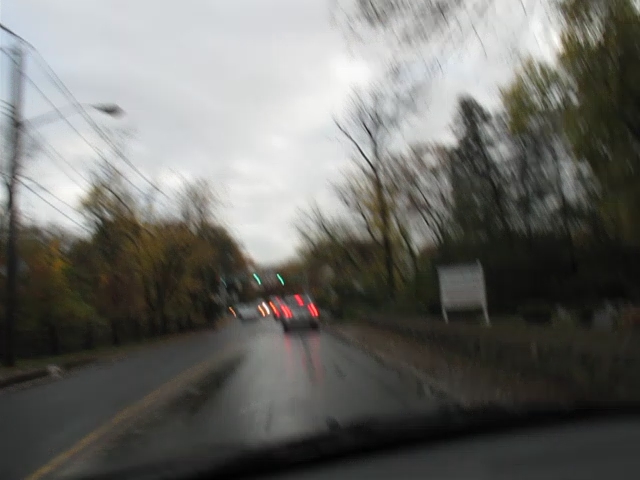In the foreground, on the left side of the image, stands a telephone pole with wires extending horizontally across the scene. Nearby, a lamppost juts out of the wet, reflective black asphalt of the street, accentuated by bright yellow lines stretching into the distance. A car is visible, its red taillights glowing vividly. In the background, a green traffic light is illuminated, offering a sense of depth and context to the urban setting. On the right side of the image, an abundance of trees with lush leaves provides a natural contrast to the man-made elements. A white sign is partially visible, adding to the suburban feel of the scene, while numerous branches and additional trees frame the leftmost edge of the composition.